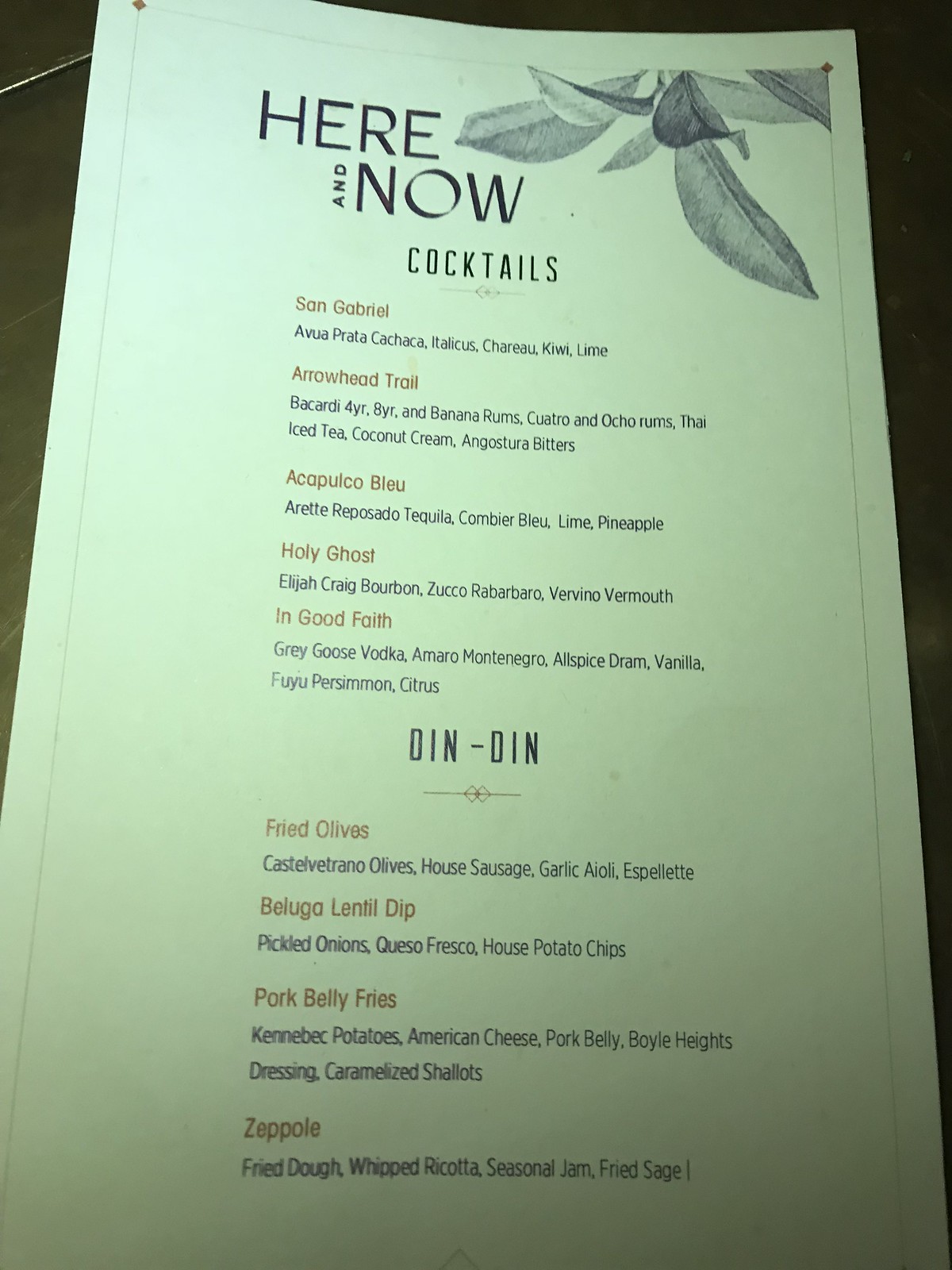The image captures a dimly lit restaurant or bar menu, taken with a flash that highlights its textures and colors. The menu, printed on beige paper with a delicate white margin around the edges, rests atop a black tabletop. Decorative leaf artwork adorns the upper right-hand corner, adding a touch of elegance to the layout. The photograph has a greenish hue, possibly due to the lighting conditions. 

The menu features two primary sections: "Cocktails" and "Din-Din." 

**Cocktails**:
- **San Gabriel**: Ingredients listed below.
- **Arrowhead Trail**: Ingredients listed below.
- **Acapulco Blue**: Ingredients listed below.
- **Holy Ghost**: Ingredients listed below.
- **In Good Faith**: Ingredients listed below.

**Din-Din**:
- **Fried Olives**: Ingredients listed below.
- **Beluga Lentil Dip**: Ingredients listed below.
- **Pork Belly Fries**: Ingredients listed below.
- **Zeppoli**: Ingredients listed below.

Overall, the menu presentation and the detailed flash-lit photograph provide a thorough glimpse into the establishment's offerings amidst an intimate setting.